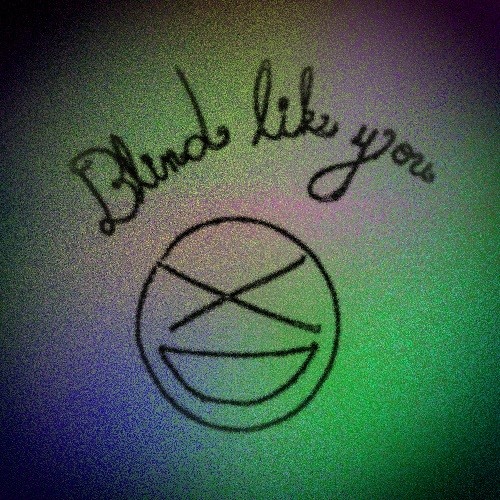The image is a square photograph with a grainy texture and a vignette effect, making the corners dark. The background is an abstract blend of greenish, bluish, and pinkish hues, with richer concentrations of yellow and green at the top, and purple and blue transitioning from the bottom left to the upper right. Centered within the image, just below the top edge, is a line of black cursive text that curves gracefully, reading "blind like you." Below this text is a simple stick-figure drawing resembling an emoticon. The figure's head features a large, open, smiling mouth. However, instead of eyes, there is a prominent X across the upper portion of the head, symbolizing blindness. The image combines the whimsical nature of a smiley face with a poignant message, creating a striking visual effect.